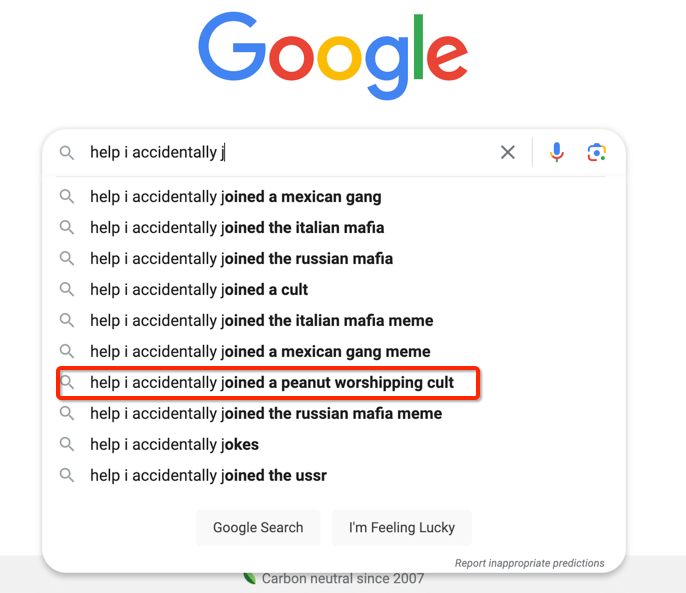The image is a screenshot of a Google search page where someone has typed "help, I accidentally J" in the search bar. As they type, the autocomplete suggestions appear below. The partially completed search prompt generates an assortment of humorous and bizarre options:

1. Help, I accidentally joined a Mexican gang
2. Help, I accidentally joined the Italian mafia
3. Help, I accidentally joined the Russian mafia
4. Help, I accidentally joined a cult
5. Help, I accidentally joined the Italian mafia meme
6. Help, I accidentally joined a Mexican gang meme
7. Help, I accidentally joined a peanut worshiping cult (this option is highlighted with a red box for its absurdity)
8. Help, I accidentally joined the Russian mafia meme
9. Help, I accidentally jokes
10. Help, I accidentally joined the USSR

The page is a typical Google search interface, complete with an "X" button to clear the search query, a microphone icon for voice input, and a camera icon for image search. At the bottom of the search box, there are two prominent buttons: "Google Search" and "I'm Feeling Lucky." The screenshot perfectly captures the quirks of Google's autocomplete feature and its sometimes strange sense of humor.